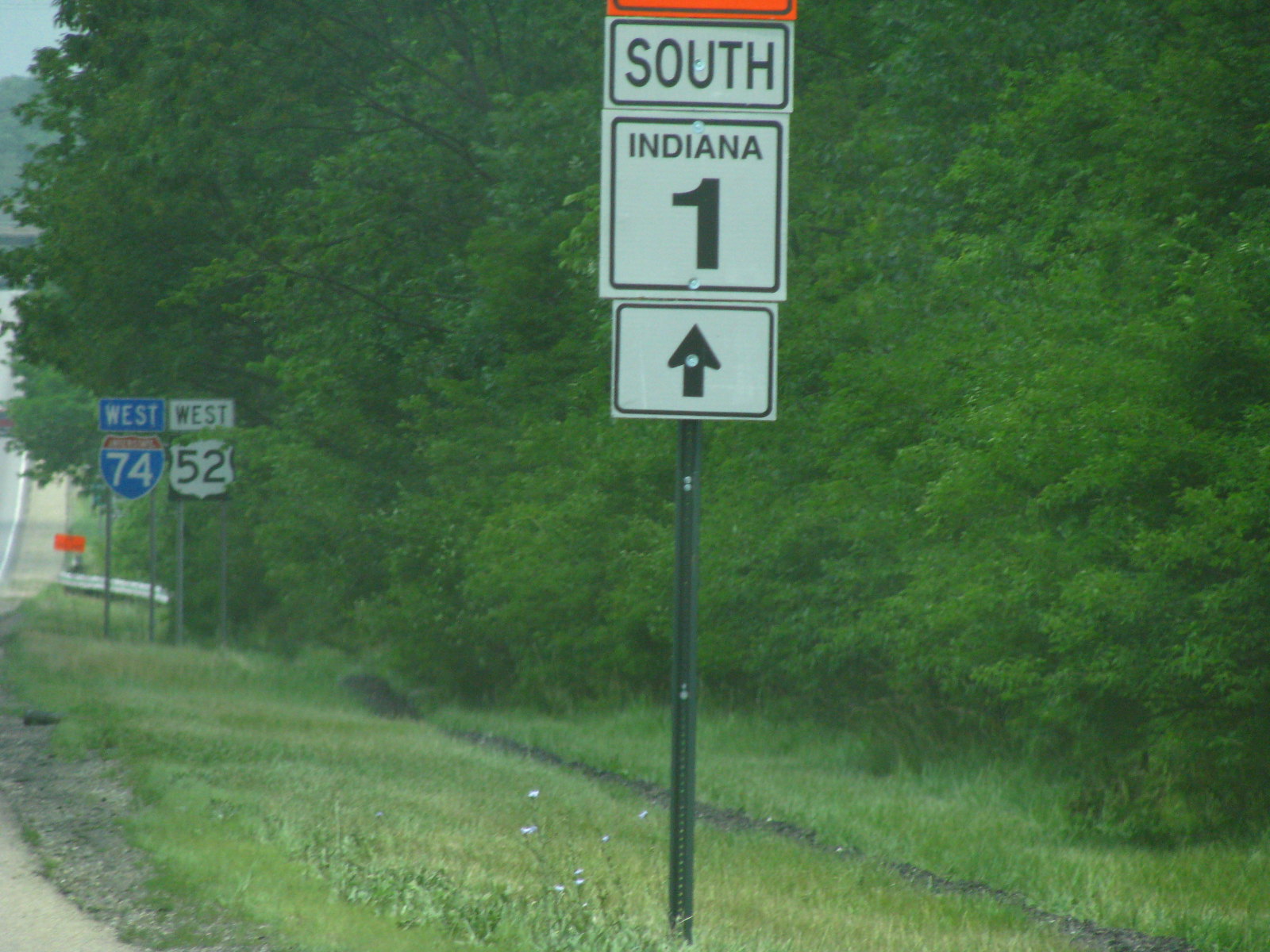The daytime photograph captures the serene side of a road bordered by a lush, green shoulder lined with grass and dotted with tiny white wildflowers, indicating a warm climate. Trees densely populate the right side of the image, creating a natural, leafy frame. At the center, a green street sign points straight ahead and reads "South Indiana 1," accompanied by a blue sign further along that indicates "West Interstate 74." To the right, a white street sign with black text directs towards "West Highway 52," adding to the intricate network of directions amidst the verdant backdrop.